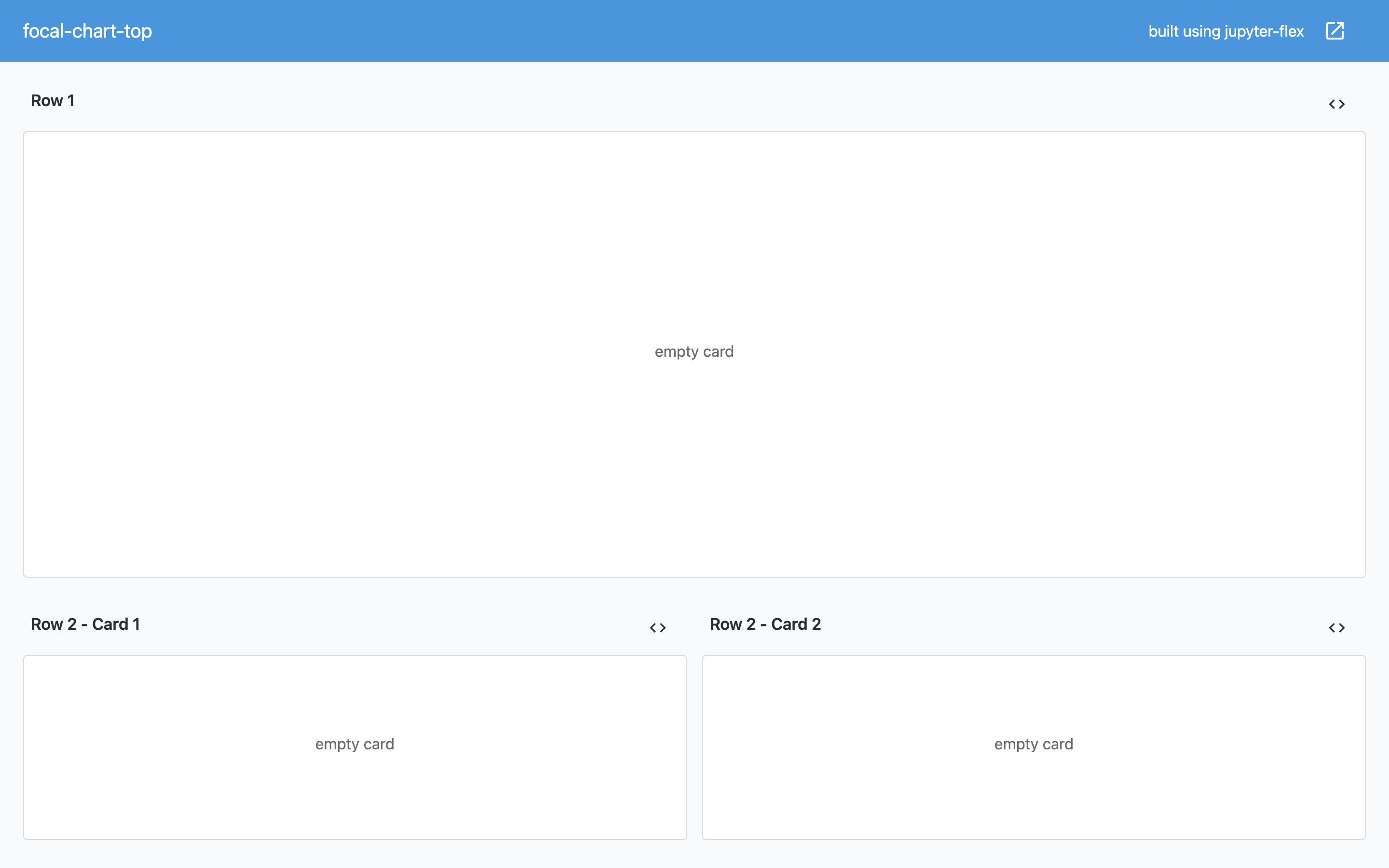This image features a design element set against a muted gray background. Central to the composition is a striking blue rectangle. Complementing the blue rectangle is a segmented, circular "spoke" chart, which is labeled "Bullet," created using the Jupiter Flex software. Within the image, there is also a white square with a diagonal arrow pointing up and to the right. Below the chart, a structured grid displays various interactive elements. In 'Row 1,' there are left and right navigation arrows accompanied by a white rectangle labeled "Empty Card." 'Row 2' mirrors this arrangement, presenting two cards labeled "Card 1" and "Card 2," each enclosed within a white rectangle, accompanied by left and right navigation arrows, and also labeled "Empty Card."